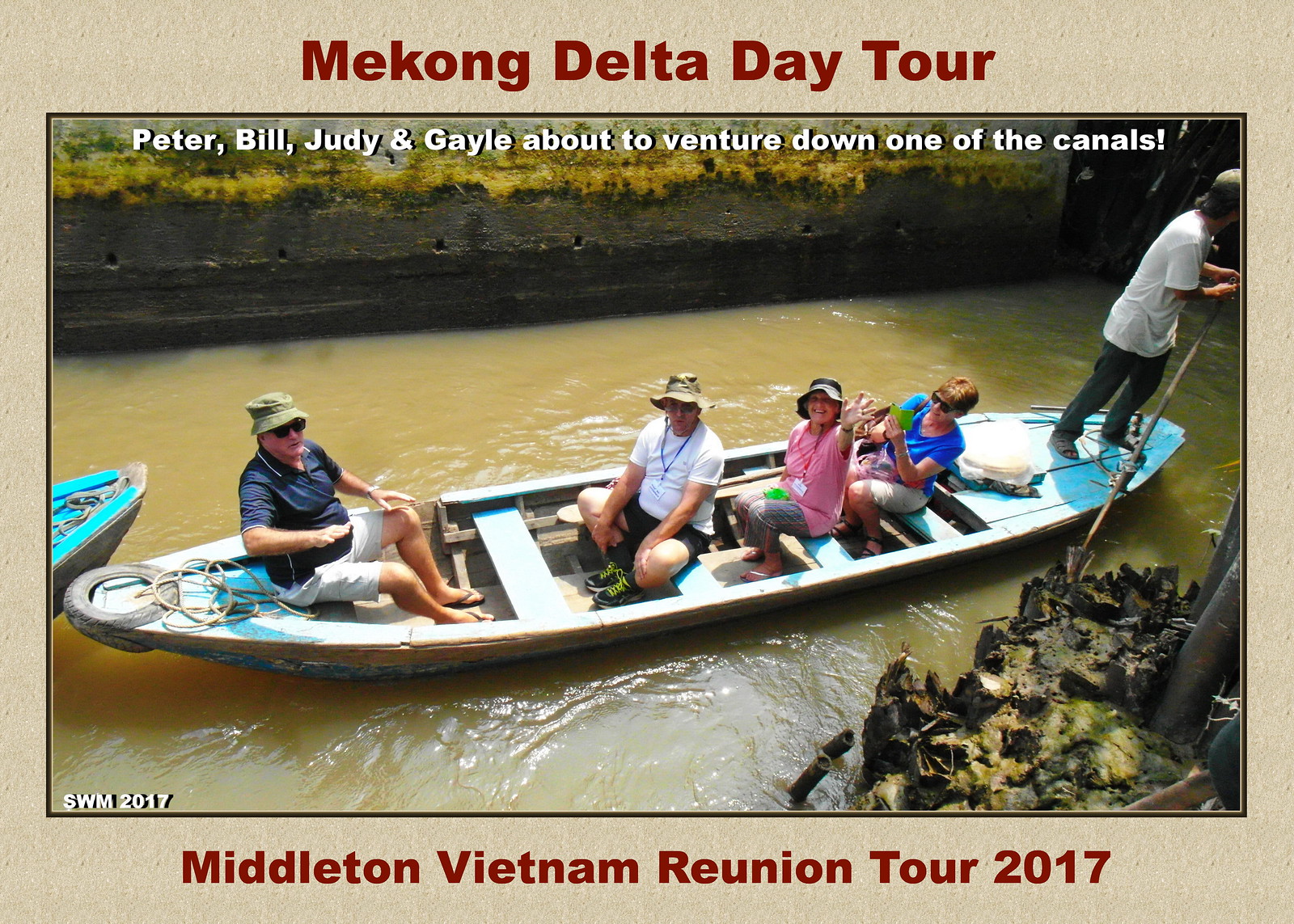In this vibrant outdoor daytime photograph, four middle-aged, white individuals, identified as Peter, Bill, Judy, and Gail, are seated in a pale gray boat navigating a muddy canal possibly in Vietnam. The men wear sun hats and are dressed in casual attire; one man sports a blue shirt with beige shorts and sandals, while the other wears a white shirt with a blue lanyard, black shorts, and dark sneakers. Judy is seen in a pink shirt with a red lanyard, striped pants, and sandals, whereas Gail wears sunglasses, a blue shirt, and khaki pants. Standing at the front of the boat, guiding it with a pole, is an Asian man in a white t-shirt and dark pants. A blue boat trails behind them. The image features text over a light brown, slide-like background with dark red captions. The top reads "Mekong Delta Day Tour," followed by "Peter, Bill, Judy, and Gail about to venture down one of the canals." The bottom text announces "Middleton Vietnam Reunion Tour 2017," with the initials "SWM" and "2017" in the bottom left corner. In the foreground, some rocks can be seen, adding depth to the scene dominated by the concrete wall and reflective, murky waters of the canal.